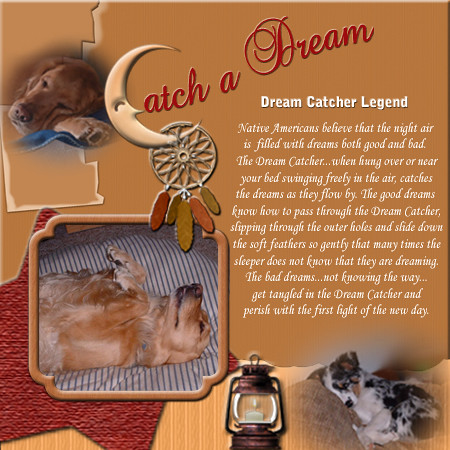A digitally created collage features multiple dog pictures and elements centered around the theme of dreamcatchers and Native American legends. At the center of the poster, in dark red cursive lettering, it says "Catch a Dream," with part of the lettering forming a half-moon shape with an eye and a nose. A dreamcatcher, adorned with silver webbing, hangs from the moon, cascading downwards with feathers in amber, green, and orange hues. Below this central motif, there's an artist rendition of a kerosene lantern.

On the right side, white text reads "Dreamcatcher Legend" and elaborates in smaller text: "Native Americans believe that the night air is filled with dreams both good and bad. The dreamcatcher, when hung over or near your bed, swinging freely in the air, catches the dreams as they flow by. The good dreams know how to pass through the dreamcatcher, slipping through the outer holes and sliding down the soft feathers so gently that many times the sleeper does not know that they are dreaming. The bad dreams, not knowing the way, get tangled in the dreamcatcher and perish with the first light of the new day."

At the bottom center of the poster is a picture of a puppy with a white chest, a black and white back, and brown accents on its face. Next to it on the left is a square image of a yellow dog lying on its back with its paws up, resting on a blue and white striped blanket. In the upper left corner, another dog is shown resting, with its head to the right and nose facing left, circled faintly. The overall background of the poster is predominantly tan and orange, with a pink star with rough edges in the bottom left corner, adding a whimsical touch.